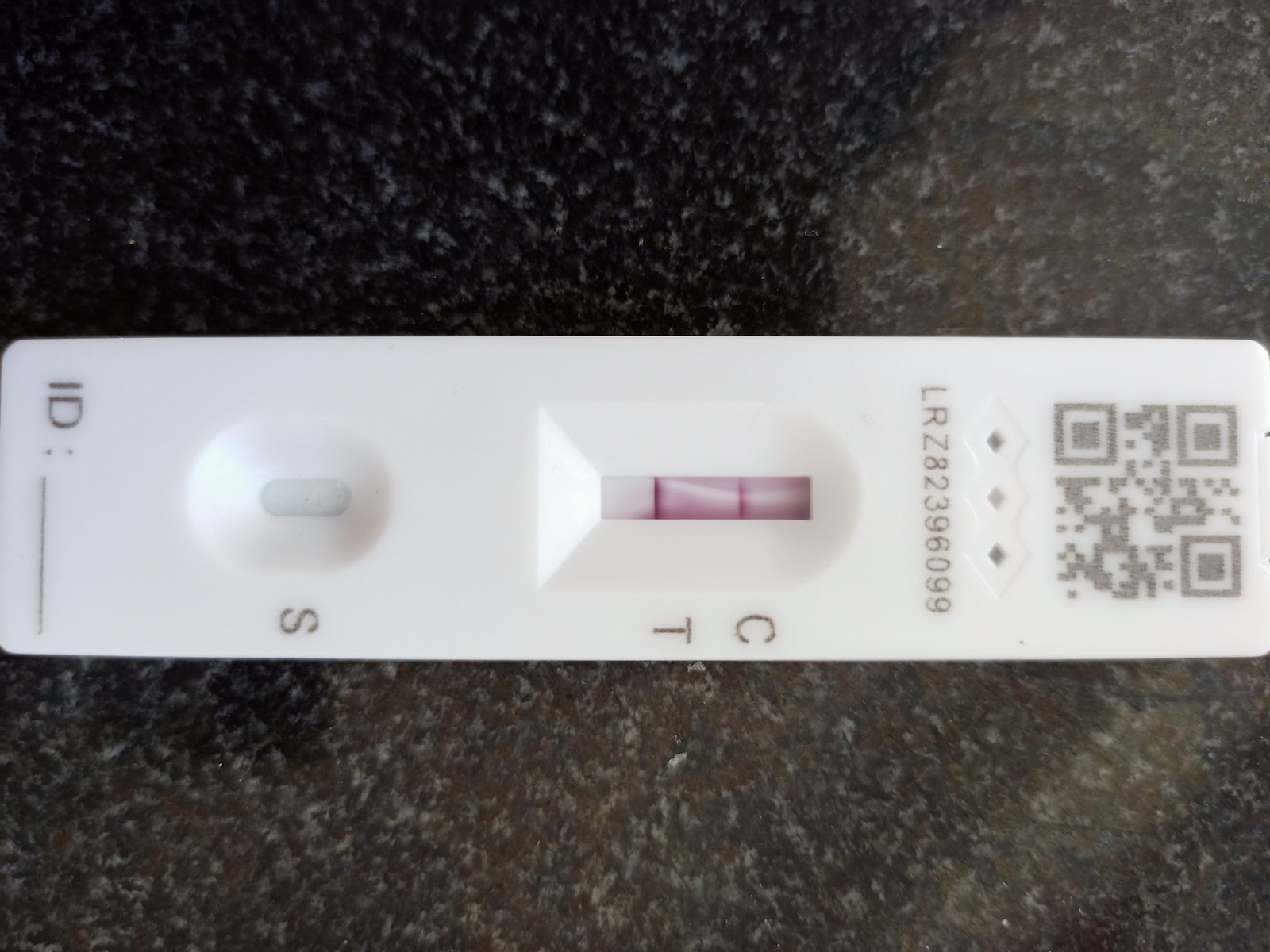Detailed Caption:

The image depicts a white electronic device, possibly a temperature gauge or a similar instrument, placed on a black and white speckled counter. At the top of the device, there is a code consisting of three squares and several digits meant to be scanned for additional information. Just below this code are three diamond-shaped symbols embedded into the white plastic, each with a small hole in the center. Beneath these symbols, there is black lettering that reads "LRZ 823 96099." To the right of this text, also in black lettering, is the abbreviation "CT."

In the middle section of the device, there is a pink area with two parallel lines. Below this pink section, the device's surface color shifts to a slightly darker shade of white and is situated within an indented crevice that resembles a door opening. At the bottom portion of the device, there is a circular element, marked with an "S" and displaying a light green hue. Lastly, the bottom edge of the device features the text "ID" followed by two colons and an underscore line, all in black.